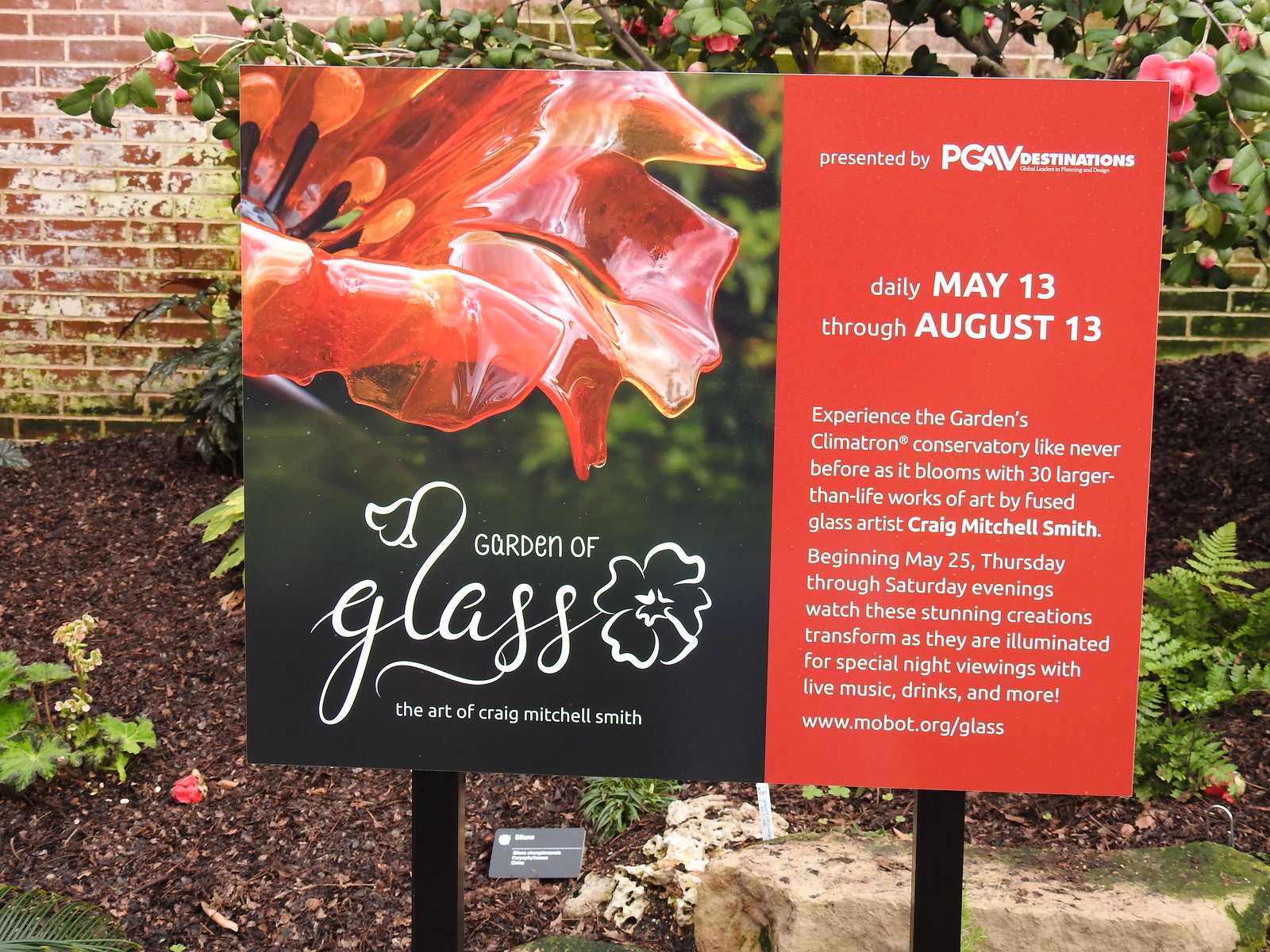The photograph shows a rectangular signboard mounted on two black posts, situated in a garden setting with soil, plants, and a brick wall in the background. The left half of the sign features an illustration of a glass-like flower with white text that reads, "Garden of Glass, the art of Craig Mitchell Smith." The right side is a red rectangle with white text providing detailed information: "Presented by PGAV Destinations, Daily May 13th through August 13th. Experience the garden's Climatron Conservatory like never before as it blooms with 30 larger-than-life works of art by fused glass artist Craig Mitchell Smith. Enjoy special night viewings with live music, drinks, and more, from Thursday to Saturday evenings starting May 25th." The sign also includes a website link, "mobot.org/glass," for additional details. The setting combines natural elements with artistic glass creations to create a unique visual experience.